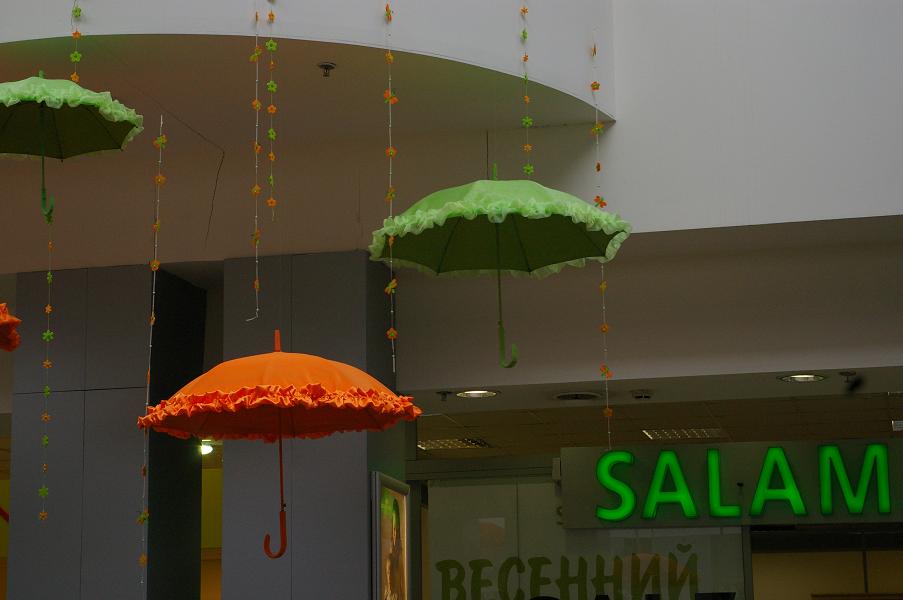In this vibrant color photograph, we see a decorative display in what appears to be a mall, possibly located in the Middle East. From the high ceiling, three exquisitely detailed umbrellas hang by thin strings adorned with small orange and green flowers. Two of the umbrellas are a bright green with ruffled edges, and one is a vivid orange with a similar frilly border. Each umbrella has a gracefully curved, hook-shaped handle that adds to the charm of the scene. Below these umbrellas, a storefront sign in bold green letters spells out "S-A-L-A-M," possibly indicating a name or greeting. Beneath it, another sign displays characters in an unfamiliar script, featuring what looks like two backward-facing Ns. The storefront and the white walls, including a visible fire sprinkler on the ceiling, suggest a clean, modern setting, characteristic of a shopping mall.